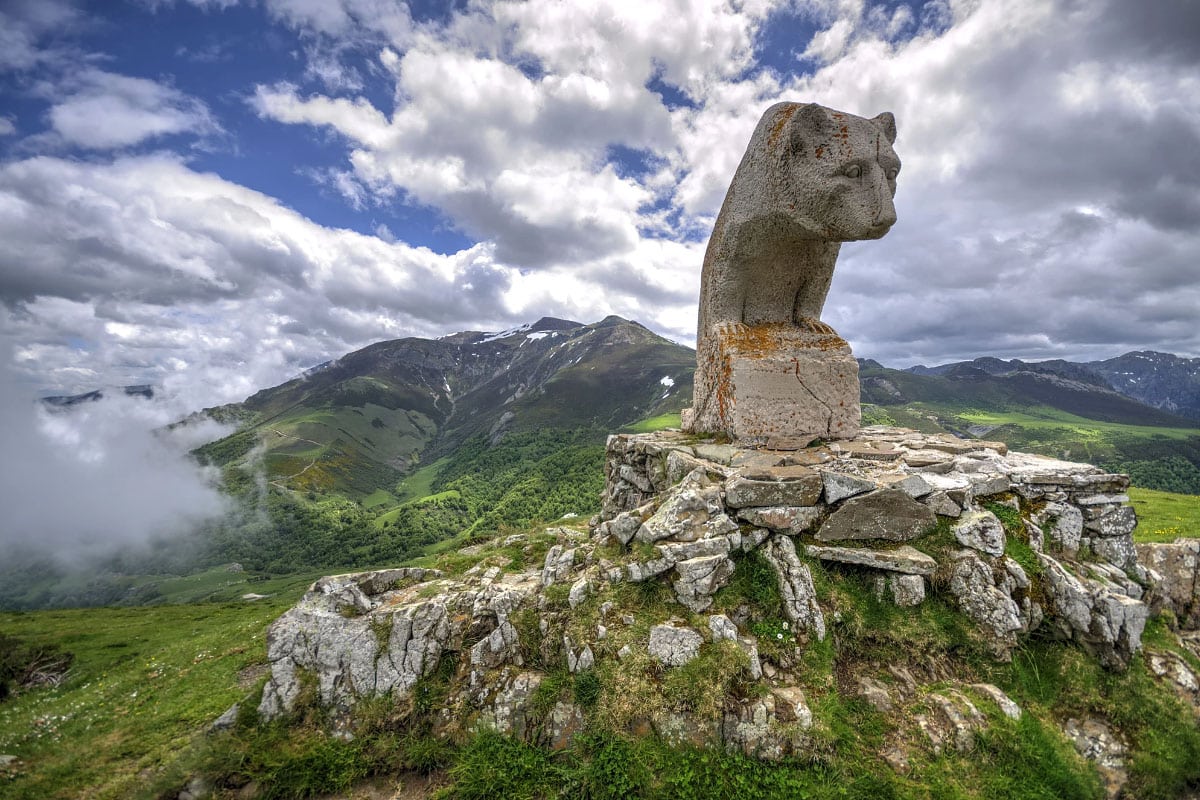The photograph captures a serene, mountainous landscape featuring a stone statue of a large feline, seemingly a cougar, poised on a rocky pedestal amidst ancient ruins. The statue, partially incomplete, gives an aged and venerable atmosphere to the scene, suggesting a historical significance. The rocky base is naturally covered in moss, blending seamlessly with the lush, green valley that stretches out below. The landscape is punctuated by towering, dark brown mountains, some capped with patches of snow. Above, a sky filled with white, fluffy clouds allows rays of sunlight to occasionally break through, casting a tranquil light over the area. A low-lying cloud hovers within a distant canyon, emphasizing the high altitude. The peaceful and untouched nature of the scene is accentuated by the absence of people or animals, making the viewer feel as if the cougar statue is vigilantly surveying the vast, undisturbed wilderness.